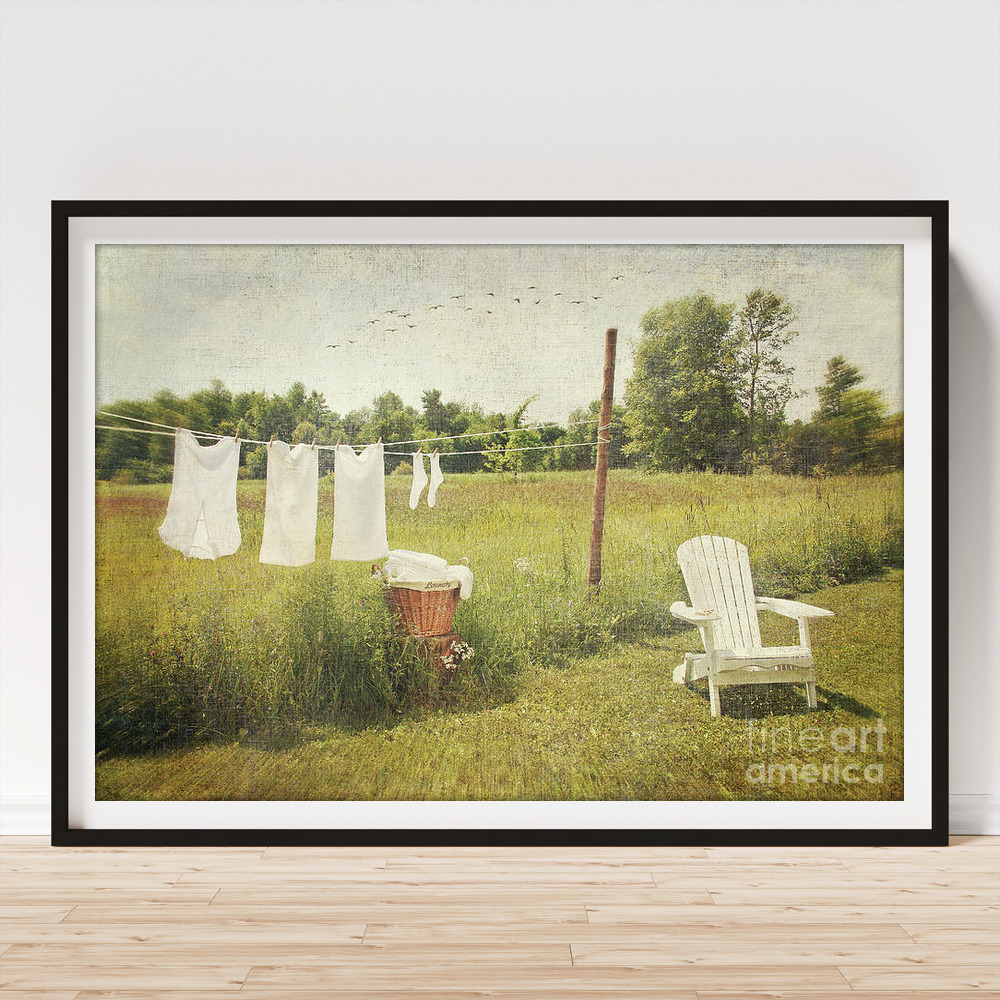The image depicts a realistic painting inside a black plastic frame with a white border, leaning against a white wall on a light brown wood plank floor. The painting portrays an outdoor scene with vibrant details. In the foreground, to the lower right, a white Adirondack chair sits on a patch of neatly trimmed green grass, transitioning into wilder, taller grasses behind it. A central wooden pole or tree branch supports a white clothesline featuring several articles of clothing: three shirts or slips, a camisole, and two white socks. Below the clothesline, there's a golden wicker basket filled with linens. In the background, the sky is mostly white and gray, scattered with birds in flight. Taller trees line the scene on the right. Near the bottom right of the painting, "Lion Art America" is inscribed.